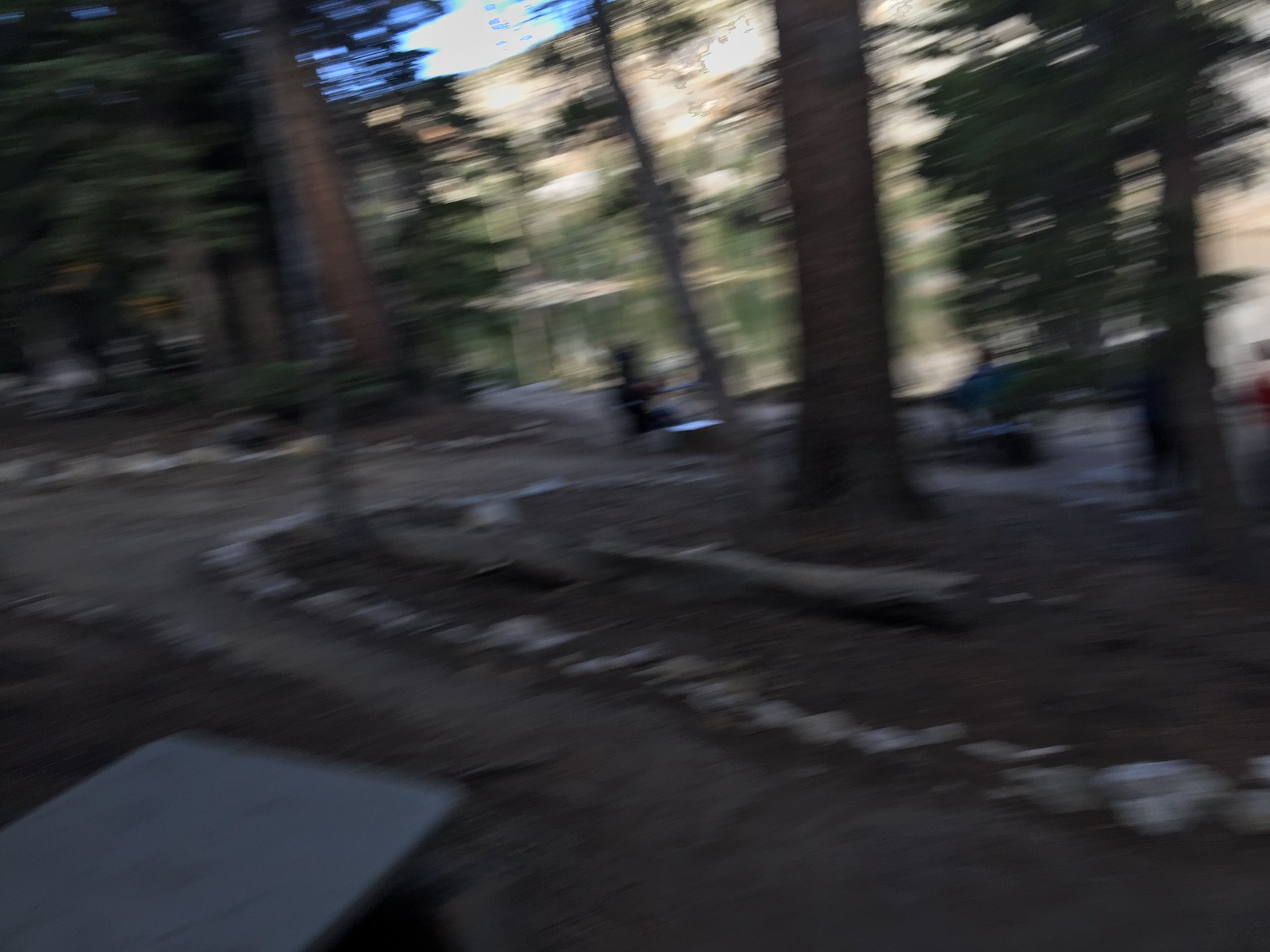This image, though blurred, depicts an outdoor scene distinguished by patches of blue sky peeking through in the top left corner, suggesting a bright day. The foreground showcases a mix of large, older trees interspersed with thinner, possibly different species, including some with vinelike characteristics. These trees appear well-established, their lush green canopies contributing to the vibrant background.

The layout of the scene suggests a planned, man-made environment resembling a natural forest setting—possibly a campground. The trees are strategically lined with stones, forming pathways of flattened dirt or gravel that meander through the area. The ground between these stone-lined pathways appears covered in darker, richer soil, possibly potting soil, enhancing the natural yet organized aesthetic. Additionally, long logs are intricately placed throughout, enhancing the intentional design and contributing to the rustic, serene ambiance of the environment.